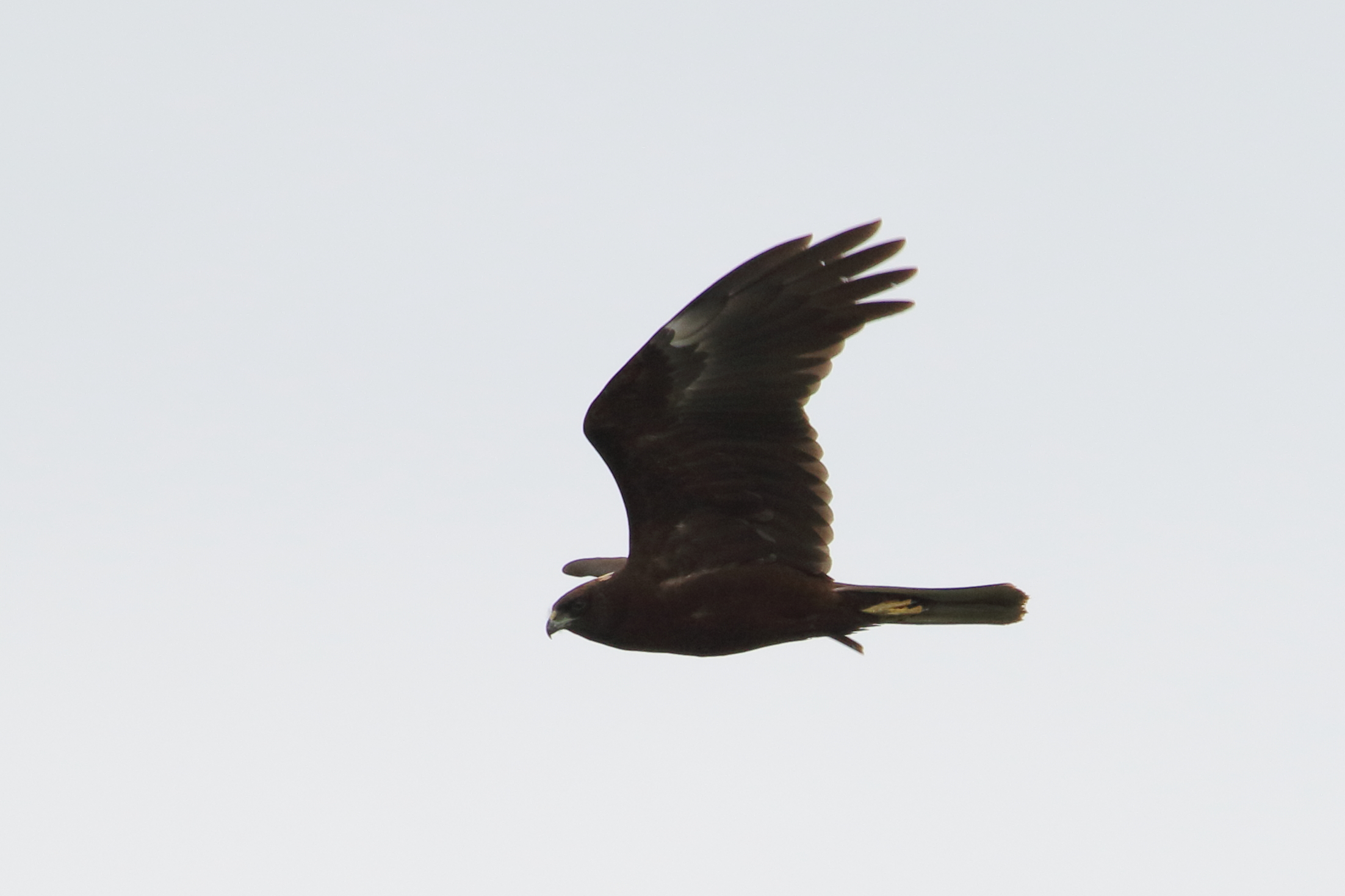A striking image captures a dark brown bird in mid-flight against a uniform light gray background, which may either be the overcast sky or another outdoor setting. Predominantly dark in color, the bird showcases a mix of black and brown plumage with lighter, possibly white or off-white, accents on its wings and near the tail feathers. This avian subject has its wings outstretched with visible feather tips and appears to be gliding horizontally towards the left side of the frame. Its tail feathers are extended horizontally, and its yellow feet are tucked against its belly, highlighting its streamlined form. The bird's small gray beak and black eyes that are barely discernible against its dark head convey an intense focus, adding a dynamic sense of movement to the otherwise minimalistic composition.